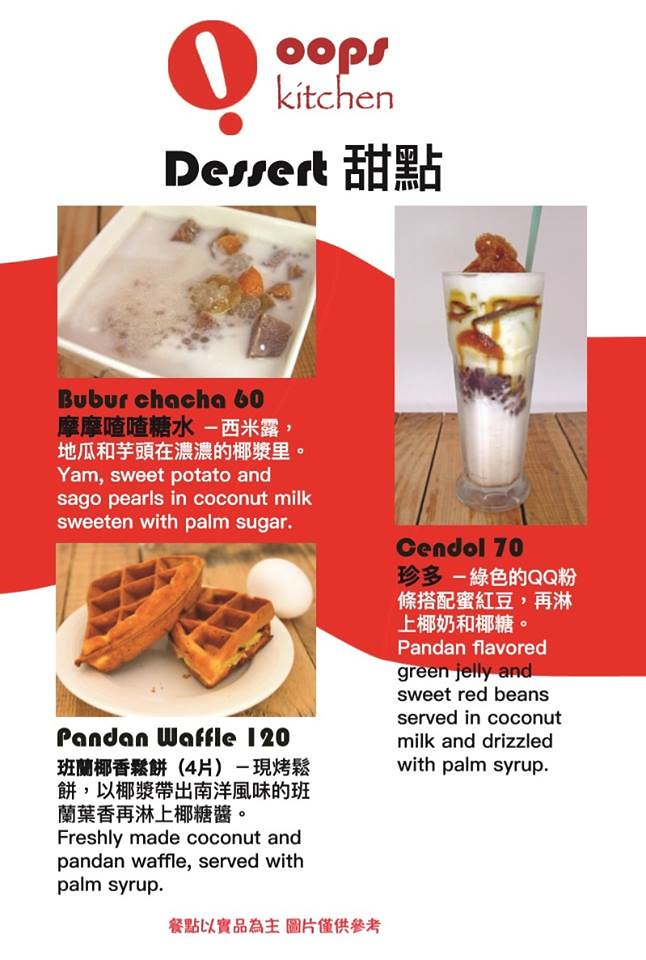The image is a detailed, three-photograph menu showcasing a selection of desserts from "Oops Kitchen." At the top, "Oops Kitchen" is prominently displayed in bold red font, accompanied by the word "dessert" in black text and two Chinese characters. To the left of the text is a red circle with a white exclamation point.

The left photograph features a dessert named "Bubur Cha Cha" priced at 60, presented in a square white bowl viewed from above. Below the name, there are Chinese characters and a detailed description reading, "Yam, Sweet Potato, and Sago Pearls in Coconut Milk, Sweetened with Palm Sugar."

The middle photograph showcases a sundae glass containing a white, milky substance and a blue straw, labeled "Cendol" at a price of 70. Beneath the name, the description includes Chinese script.

The right photograph depicts "Pandan Waffle" priced at 120, with two wedges of a waffle and a white egg behind them, served on a round white plate. The caption includes additional Chinese characters below the name.

The style of the menu merges photographic realism with graphic design and typography, providing a clear and visually appealing representation of the desserts offered.